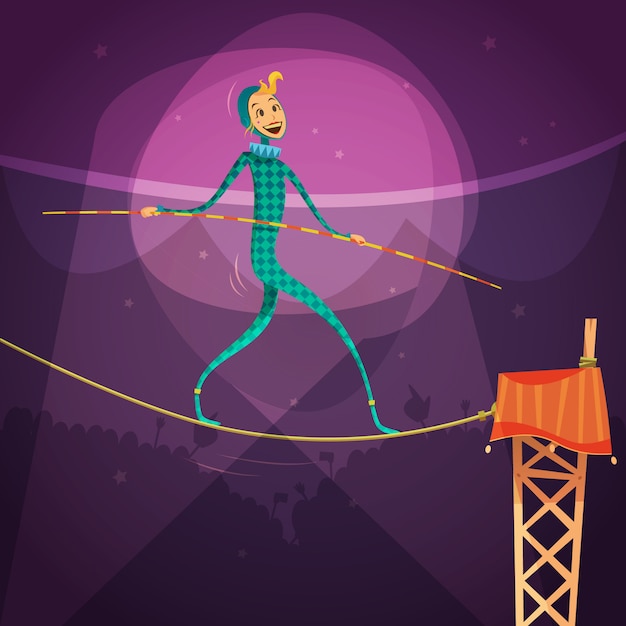The image is a whimsical, 2D illustration of a tightrope performance, possibly part of a circus act. In the foreground, a woman balances confidently on a yellow tightrope, extending from an elevated tower on the right side to the left of the image. She wears a form-fitting green outfit adorned with dark green diamonds, complemented by a blue collar. A green mask covers her head, with wisps of golden hair peeking out from beneath her hood. Her legs appear as thin, bendy lines; her arms hold a long balancing pole, colored red and yellow, with barely noticeable hands gripping it. She smiles broadly, undaunted and joyful, as light shines on her vibrant figure and the purple, curtain-like background. The entire scene exudes a playful, cartoonish charm.